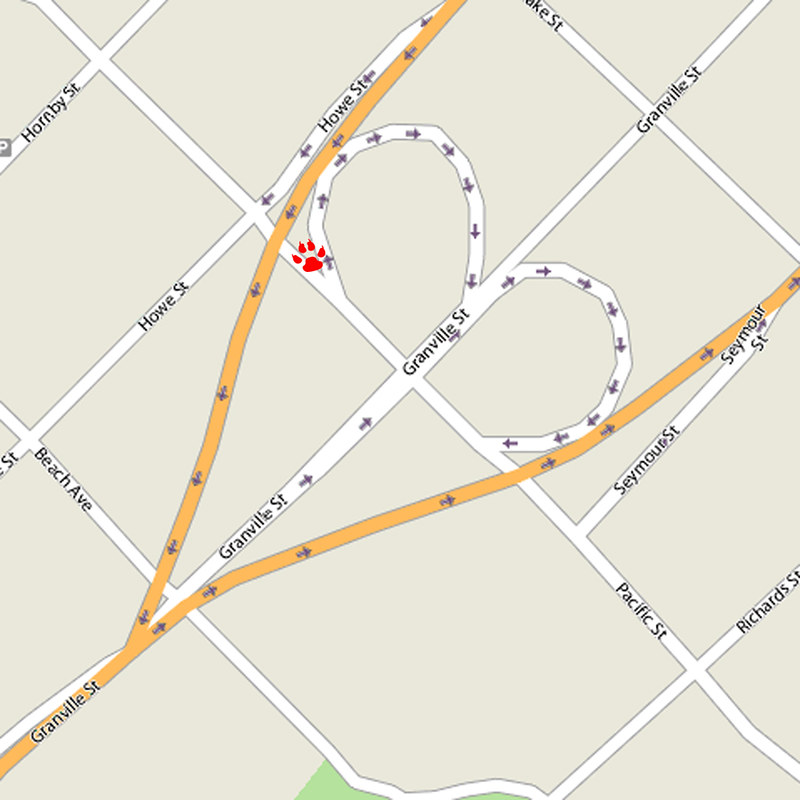The image features a detailed map with a light brown background that takes up the entirety of the image. Dominating the composition is Granville Street, highlighted in yellow, which starts from the lower left and forks into two directions towards the upper right and far right, both still labeled as Granville Street. Surrounding this main street, a variety of other roads such as Pacific Street, Richard Street, Beach Avenue, Howe Street, Hornby Street, and Seymour Street are clearly marked against a tan and gray backdrop, with street names written in black font. The map also contains color accents of tan, white, gray, black, orange, and green, and notably includes a red paw print on one fork of Granville Street. The grid-like pattern of the streets suggests this is a city map, presented as a screenshot from a computer.